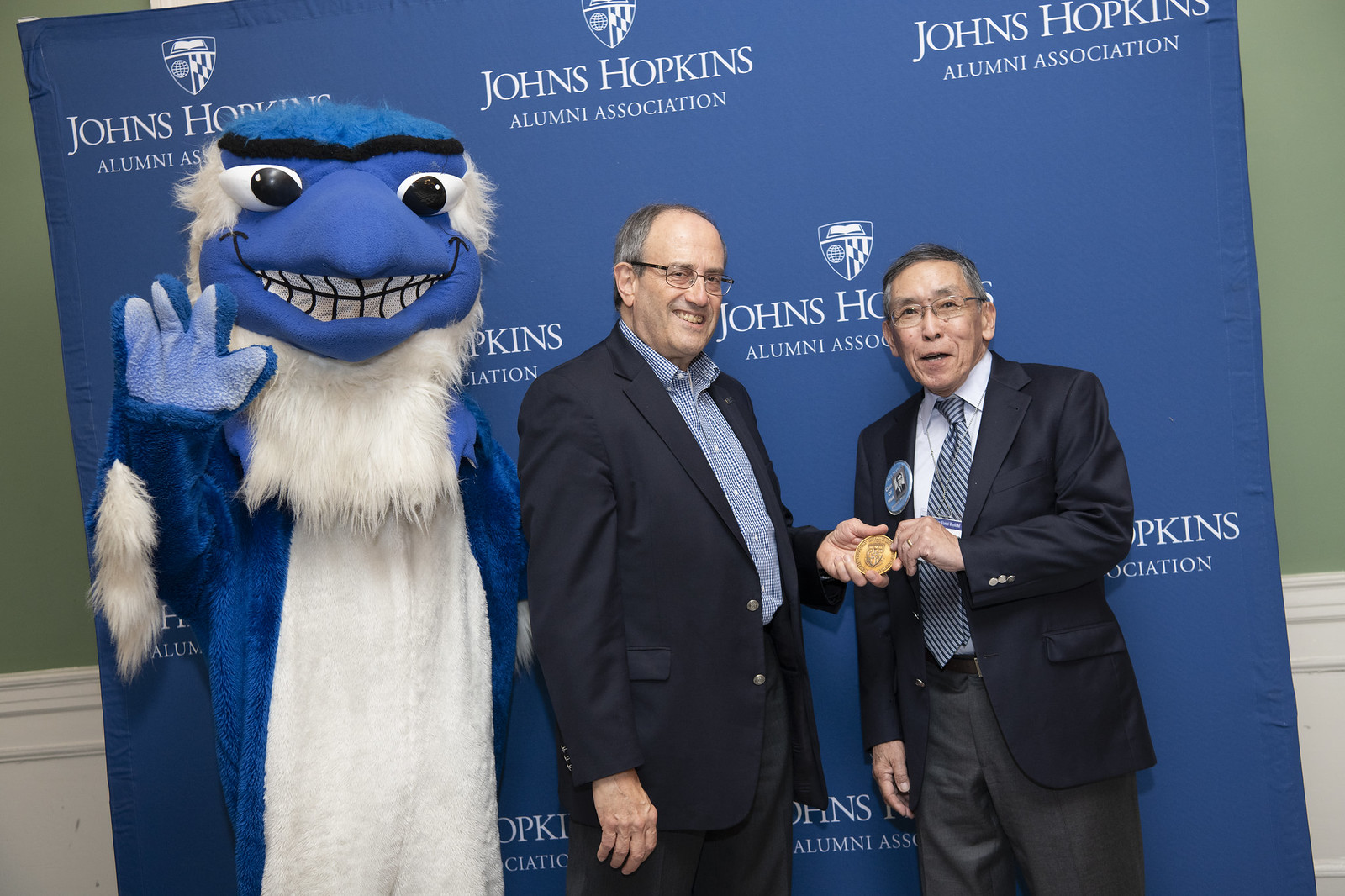In this landscape color photograph, we see a clear and bright interior scene featuring three central figures—two men and a mascot—posing together for the camera. The men, appearing to be an American and an Asian, are standing close together, smiling warmly as they hold a round emblem between them. The man on the left, wearing a black blazer with a blue shirt and wire-rimmed glasses, has a receding hairline and is holding a gold shield badge. The man on the right, dressed in a dark blazer, blue shirt, blue tie, and gray pants, has gray hair and Asian features. 

To their left, a lively bluebird mascot with a blue beak, white belly fur, and blue paws waves cheerfully at the camera. Behind them, a distinct blue banner with white lettering reads "Johns Hopkins Alumni Association," repeating multiple times and adding a formal touch to the setting. The backdrop includes green and white colored walls with molding visible, suggesting the scene is set indoors at an alumni meetup event. 

The image is crisply detailed, capturing the joyous moment with natural light enhancing the clarity and colors of the setting.